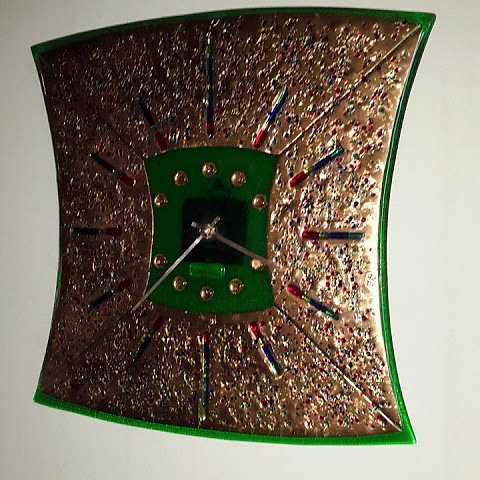This image showcases an ornate analog clock mounted on a light-colored wall. The clock, which appears to be square but is slightly distorted, features a bronze face embedded with colorful specks or gems. These embellishments line the face of the clock, denoting each hour with vibrant colors ranging from red, yellow or white, to blue, and possibly green. The 12 and 6 o'clock positions are marked with longer lines, while shorter lines mark the other hours.

At the center of the clock's face is a green, distorted square that echoes the overall shape of the clock. Within this central square, ten gems are arranged in an arch both above and below the clock hands. Just below the center, there is a smaller, brighter green rectangle, the purpose of which is unclear. The clock hands are gold or bronze, with the hour hand pointing just before the four and the minute hand between the seven and the eight, indicating the time as approximately 3:38 p.m.